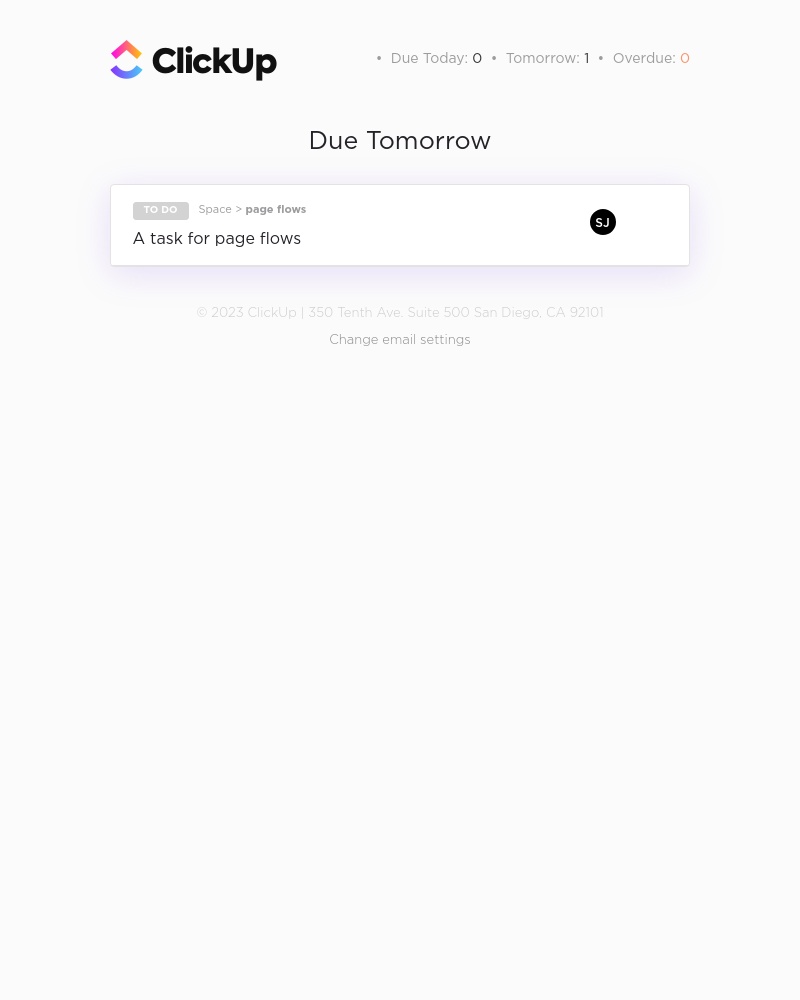The image displays a tablet screen showcasing the ClickUp productivity app. Within the interface, there's a prominent notification indicating a task with the title "Page Flows" that is due tomorrow. This reminder appears in a dialog box, ensuring the user is aware of the impending deadline. The task seemingly involves a person or entity labeled as "5J" or "SJ." 

In addition, the screen provides details such as the address of ClickUp's headquarters: 350 10th Avenue, Suite 500, San Diego, California, 92101. There is also an option to change email settings.

The overall background of the app is a light beige, with a clean layout comprising primarily black and gray text. Notable accents include a colorful ClickUp logo featuring red, orange, and blue, contributing to the app's visual appeal. The interface indicates that there are currently no tasks due today and no overdue tasks, emphasizing the single task due tomorrow.